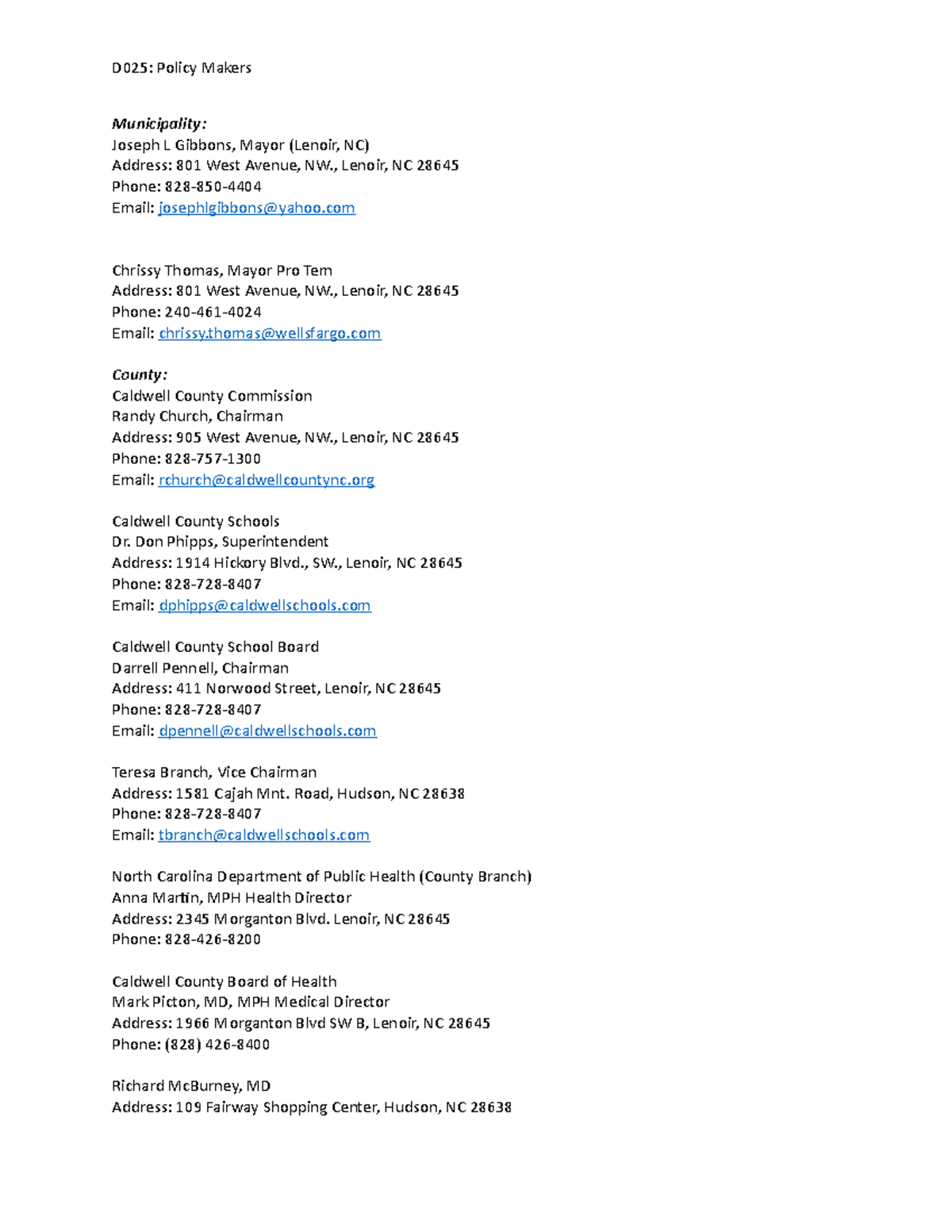This is a meticulously detailed screenshot capturing a list of policymakers, featuring their contact information. The image has a plain white background. The content is organized into various sections starting with "D025 Policymakers" in bold text at the top.

### Municipality
1. **Joseph L. Gibbons, Mayor (Lenoir, NC)**
   - **Address:** 801 West Avenue NW, Lenoir, NC 28645
   - **Phone Number:** 828-850-4404
   - **Email:** JosephLGibbons@yahoo.com

2. **Chrissy Thomas, Mayor Pro-Tem**
   - **Address:** Same as the Mayor
   - **Phone Number:** 240-461-4024
   - **Email:** Chrissy.Thomas@WellsFargo.com

### County (Highlighted Section)
1. **Caldwell County Commission**
   - **Randy Church, Chairman**
     - **Address:** 905 West Avenue NW, Lenoir, NC 28645
     - **Phone Number:** 828-757-1300
     - **Email:** RChurch@CaldwellCountyNC.org

2. **Caldwell County Schools**
   - **Dr. Don Phipps, Superintendent**
     - **Address:** 1914 Hickory Boulevard SW, Lenoir, NC 28645
     - **Phone Number:** 828-727-8407
     - **Email:** DPhipps@CaldwellSchools.com

3. **Caldwell County School Board**
   - **Darrell Pennell, Chairman**
     - **Address:** 411 Norwood Street, Lenoir, NC 28645
     - **Phone Number:** 828-728-8407
     - **Email:** DPennell@CaldwellSchools.com

   - **Teresa Branch, Vice Chairman**
     - **Address:** 1581 Cajah Mountain Road, Hudson, NC 28638
     - **Phone Number:** 828-728-8407
     - **Email:** TBranch@CaldwellSchools.com

4. **North Carolina Department of Public Health (County Branch)**
   - **Anna Martin, MPH, Health Director**
     - **Address:** 2345 Morganton Boulevard, Lenoir, NC 28645
     - **Phone Number:** 828-426-8200

5. **Caldwell County Board of Health**
   - **Mark Picton, MD, MPH, Medical Director**
     - **Address:** 1966 Morganton Boulevard SWB, Lenoir, NC 28645
     - **Phone Number:** 828-426-8400

6. **Richard McBurney, MD**
   - **Address:** 109 Fairway Shopping Center, Hudson, NC 28638

This curated list provides essential contact details, including addresses, phone numbers, and emails, for the pertinent officials in Caldwell County, NC, ensuring ease of access and communication for public inquiries and engagements.